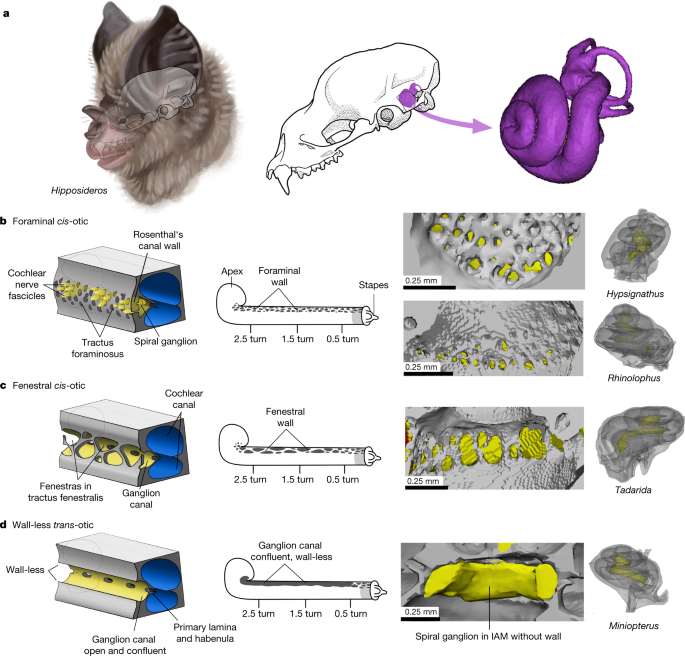This detailed infographic from a biology textbook illustrates a bat-like mammal called Hipposideros, characterized by its elongated, oblong skull and light brown fur. The central skull image prominently displays a purple gland within, possibly part of the cochlear system, essential for the bat's echolocation. Surrounding the main diagram are labeled sections B, C, and D, providing intricate cross-section designs and microscopic photos that delve into various anatomical features, such as the cochlear nerve, spiral ganglion, and Rosenthal's canal. Measurements and terms like "formineal cystostic," "stapes," and "hypocinnamus" are meticulously noted, emphasizing details of the bat’s auditory structures. This scientific and comprehensive visual representation offers a deep dive into the bat’s anatomy and hearing mechanism.